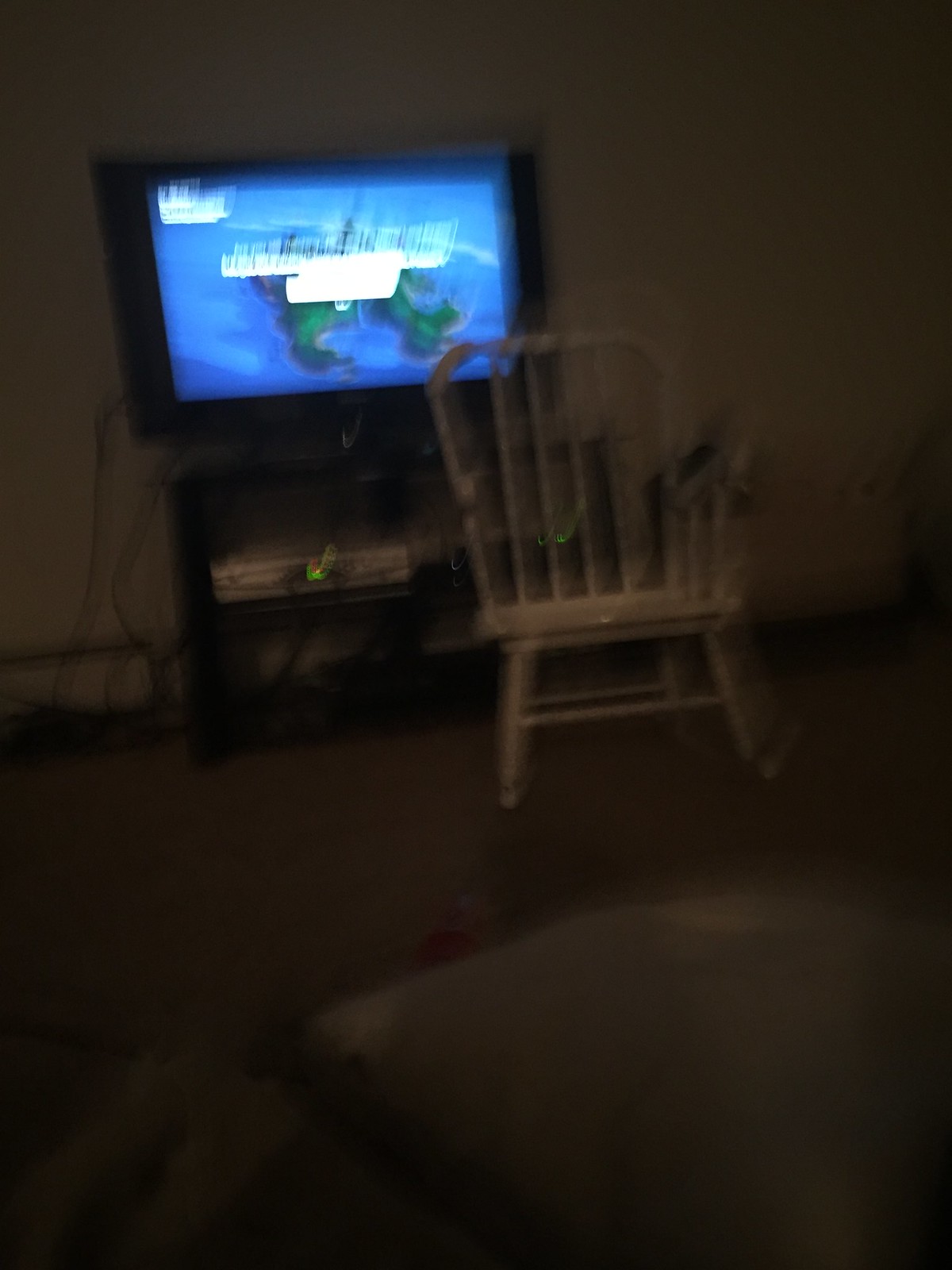A blurred, evening photograph of a dimly-lit living room, with the lights turned off. The image captures an entertainment center with a TV displaying an animated video game scene featuring an island surrounded by water, though the text on the screen is obscured due to motion blur. To the left of the TV, numerous wires are visible, possibly connecting to a VCR or game system. In front of the TV, a light-colored rocking chair, either white or gray, is positioned prominently. The picture appears to be taken from a couch, indicated by the visible pillow cushion and the edges of the beige-colored seating. The overall darkness makes it difficult to determine the precise color of the floorboards, but a noticeable red blemish, likely an object, is slightly visible past one of the cushions on the ground.